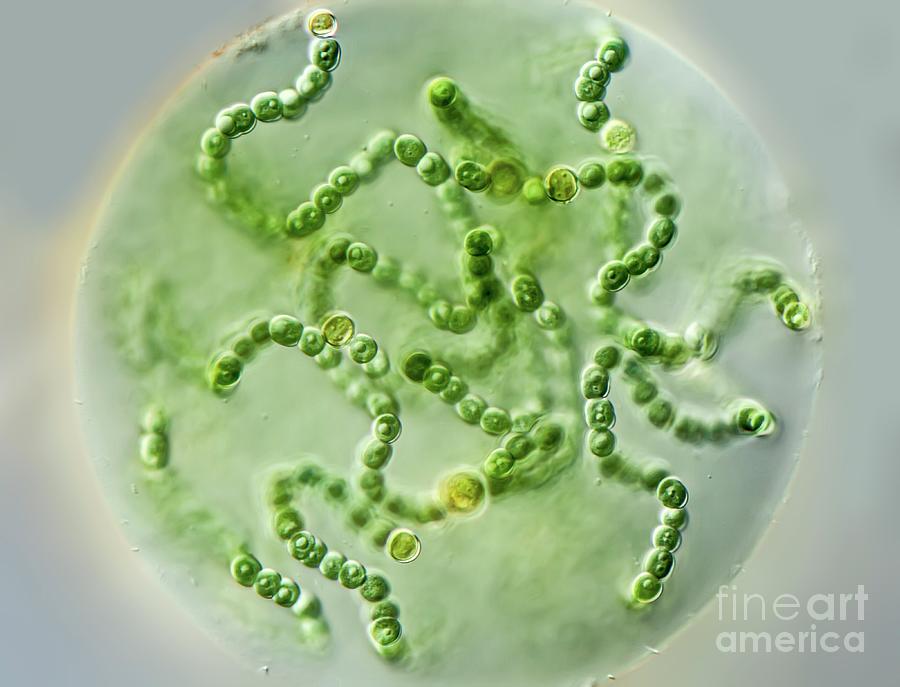This image is a highly detailed, zoomed-in view of cyanobacteria, likely captured under a microscope. The scene is framed within an off-white to gray circular area, resembling a Petri dish that occupies the majority of the image and emits a slight illumination. The microorganisms appear as long, beaded strands reminiscent of pearls on a necklace, consisting mostly of small green circles, with a sprinkling of yellowish or darker green variations. These beads vary in size, some hinting at being about pea-sized, and are distributed unevenly throughout the dish. Predominantly, four or five strands are at the forefront, standing out against approximately ten strands visible overall. The background within the Petri dish is blurred, presenting a mishmash of colors while maintaining a light gray hue that blends into the surrounding space. A watermark stating "Fine Art America" in the bottom right corner slightly bleeds into this blurred, gray background, hinting at its transparency.